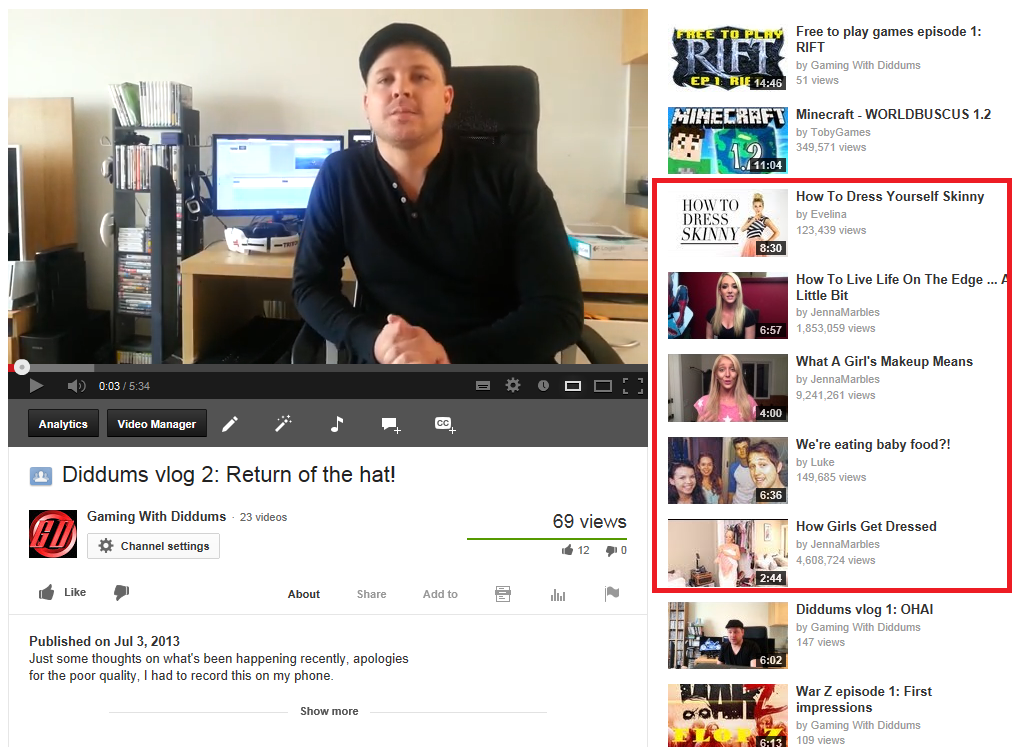This image is a screenshot from an internet search, showcasing an embedded video prominently watermarked by Photobucket, which covers the entire image, not just the video segment. The highlighted video features a man in his 30s, wearing a blue, open-necked, long-sleeved shirt, sitting in a high-backed office chair within a neat office furnished in a bamboo color scheme. The office includes a CD/DVD holder stacked with CDs, headphones, and a monitor located behind him, with possibly another cropped monitor visible to his right and a potential software package on his left.

The video interface displays key controls— a play button, an audio button, indicating the video is 3 seconds into its total duration of 5 minutes and 34 seconds, along with options for analytics, a video manager, a pencil icon, a magic wand icon, a music note icon, a conversation icon with a plus sign, and closed captions. The video's avatar is a simplistic white outline of a person on a blue background, labeled "DIDMS Vlog #2: Return of the Hat!" The channel, "Gaming with DIDMS," has 23 videos, with this particular video garnering 69 views, 12 likes, and no dislikes, and it was published on July 3rd, 2013. The video's description reads: "Just some thoughts on what's been happening recently. Apologies for the poor quality. I had to record this on my phone."

On the right side, there are nine suggested videos, the first being "Free-to-Play Games Episode 1: Rift, Minecraft, World, B-U-S-C-U-S 1.2." The next several videos are highlighted with a red rectangle and include titles like "How to Dress Yourself Skinny," "How to Live Life on the Edge a Little Bit," "What a Girl's Makeup Means," "We're Eating Baby Food!?" and "How Girls Get Dressed." Outside of the rectangle is "DIDMS Vlog 1: O-H-A-I" and "War Z Episode 1: First Impressions."

The overall visual elements underscore the amateur production quality with the watermark and in-video details, reflecting a blog-style content by a casual creator discussing personal updates alongside gaming content.